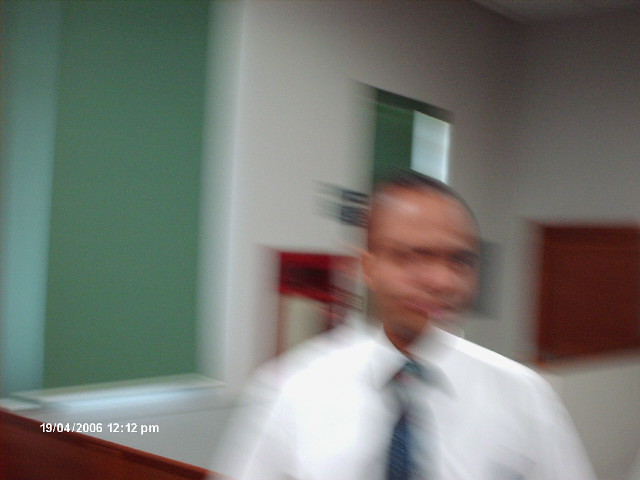This photograph, dated April 19, 2006, at 12:12 p.m., appears blurry, likely due to camera shake during capture, resulting in a doubling effect on the man's head. The man, prominent towards one side, wears a white dress shirt and a blue tie, standing against a backdrop of white walls. Two windows with green elements are visible behind him, and a wall-mounted object featuring white, black, and red colors is partly obscured by his head. Additionally, a dark-colored sign is discernible in the background. In the corners near the date stamp and on the opposite side of the image, wooden objects are visible, further detailing the scene.